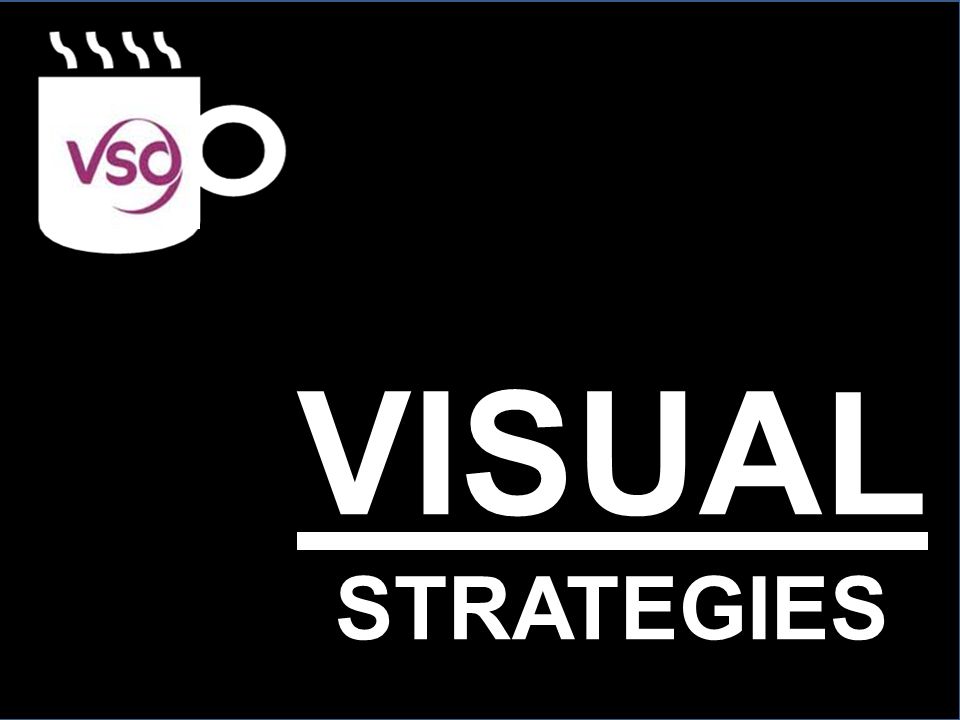The image features a solid black background displaying a stylized white coffee mug icon in the upper left corner. The mug, outlined with a circular handle positioned to the right, has steam represented by four squiggly lines rising from its top. On the front of the mug, the letters "VSO" are prominently featured in purple, with the tip of the "V" curving to encircle the "O." In the lower right corner, the words "VISUAL STRATEGIES" are displayed in large white capital letters, with "VISUAL" underlined. The word "STRATEGIES" appears in a slightly smaller font, also in white, separated by the underline. The text is presented in Arial font, adding a clean, modern touch to the image.